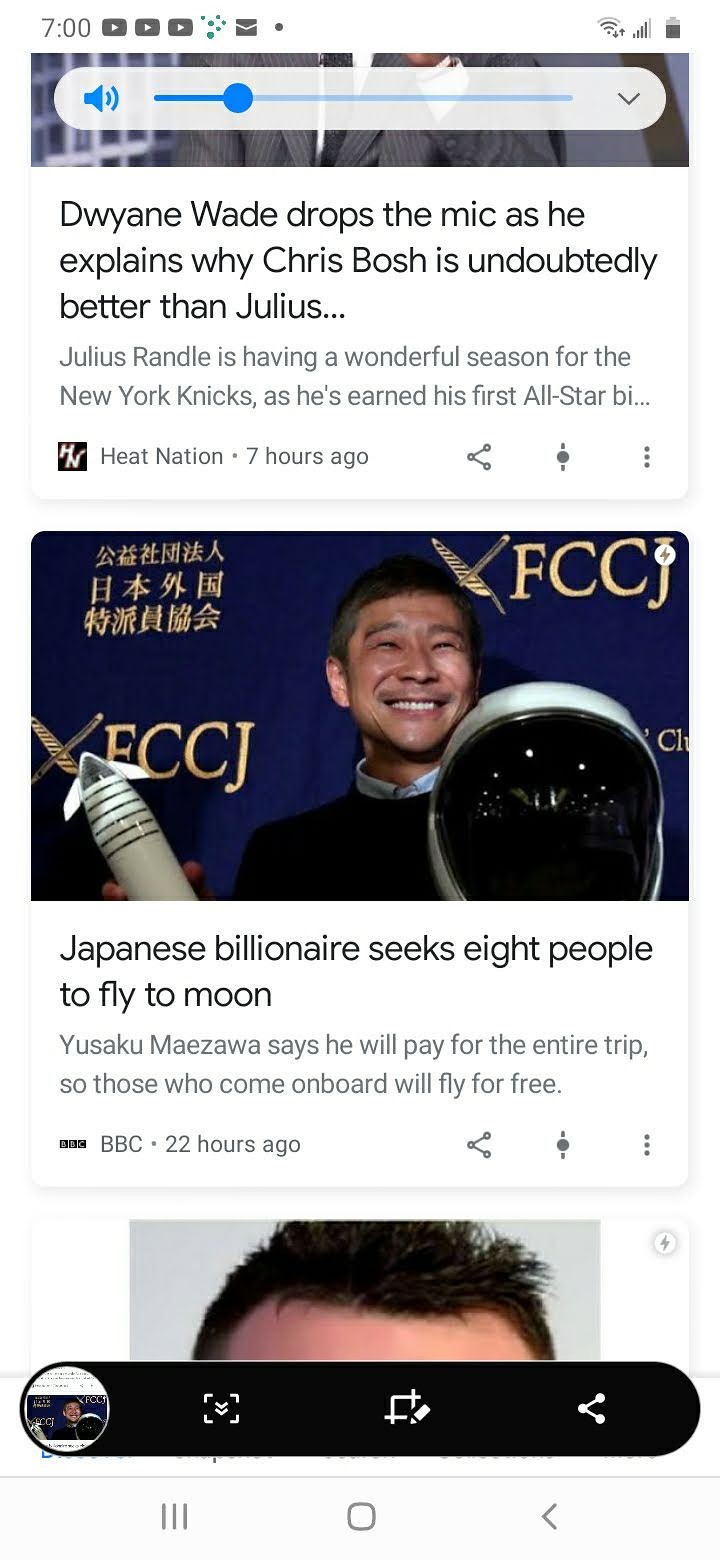This image is a screenshot of a smartphone displaying a news feed at 7 o'clock, indicated by icons typical of a non-Apple phone, including a battery at about 80% and a volume set to around 20%. At the top of the feed, there's a headline from Heat Nation posted seven hours ago: "Dwayne Wade drops the mic as he explains why Chris Bosh is undoubtedly better than Julius...". The article snippet hints that Julius Randle of the New York Knicks is having a standout season, earning his first All-Star selection. Below this, another article from the BBC posted 22 hours ago features an Asian man, identified as Japanese billionaire Yusaku Maezawa, standing in front of the letters "FCCJ" and Japanese characters. He's holding a helmet resembling a space helmet and a toy rocket. The headline reads, "Japanese billionaire seeks eight people to fly to moon," with the article noting that Maezawa will cover the entire cost of the trip, allowing selected individuals to fly for free. Both articles are presented as clickable news boxes, with a volume meter also visible above the first news article.